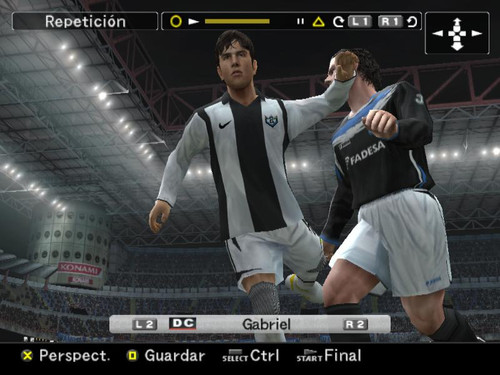The image is a detailed, likely screenshot from a video game set within a dark, digitally-rendered stadium illuminated by bright stadium lights. In the foreground, two 3D soccer characters are seen, each in motion, seemingly captured in the middle of an intense moment during a soccer match. 

The character on the left, a young man with black hair and beige skin, sports a long-sleeve white shirt with black stripes, featuring a Nike swoosh, paired with white shorts and white and gray long socks. The character on the right, who has a peachy skin tone and brown hair, wears a black shirt adorned with blue and white stripes and the word "FADESA" across the chest, coupled with white shorts and long black socks. This character appears to be running towards the left player.

Central to the image is an overlay displaying the name "Gabriel" flanked by "L2" and "R2" indicators. The bottom of the screen features a black HUD with the text "Perspect," "Guardar," "Select," "Control," "Start," and "Final" in Spanish, suggesting it's part of the game interface. The upper part of the screen reads "Repetición" in white text, likely indicating a replay mode, along with additional GUI elements such as "L1," and "R1."

In the background, the stadium's 3D crowd and the word "Konami" printed on the wall in red are distinguishable, enhancing the game's immersive atmosphere.